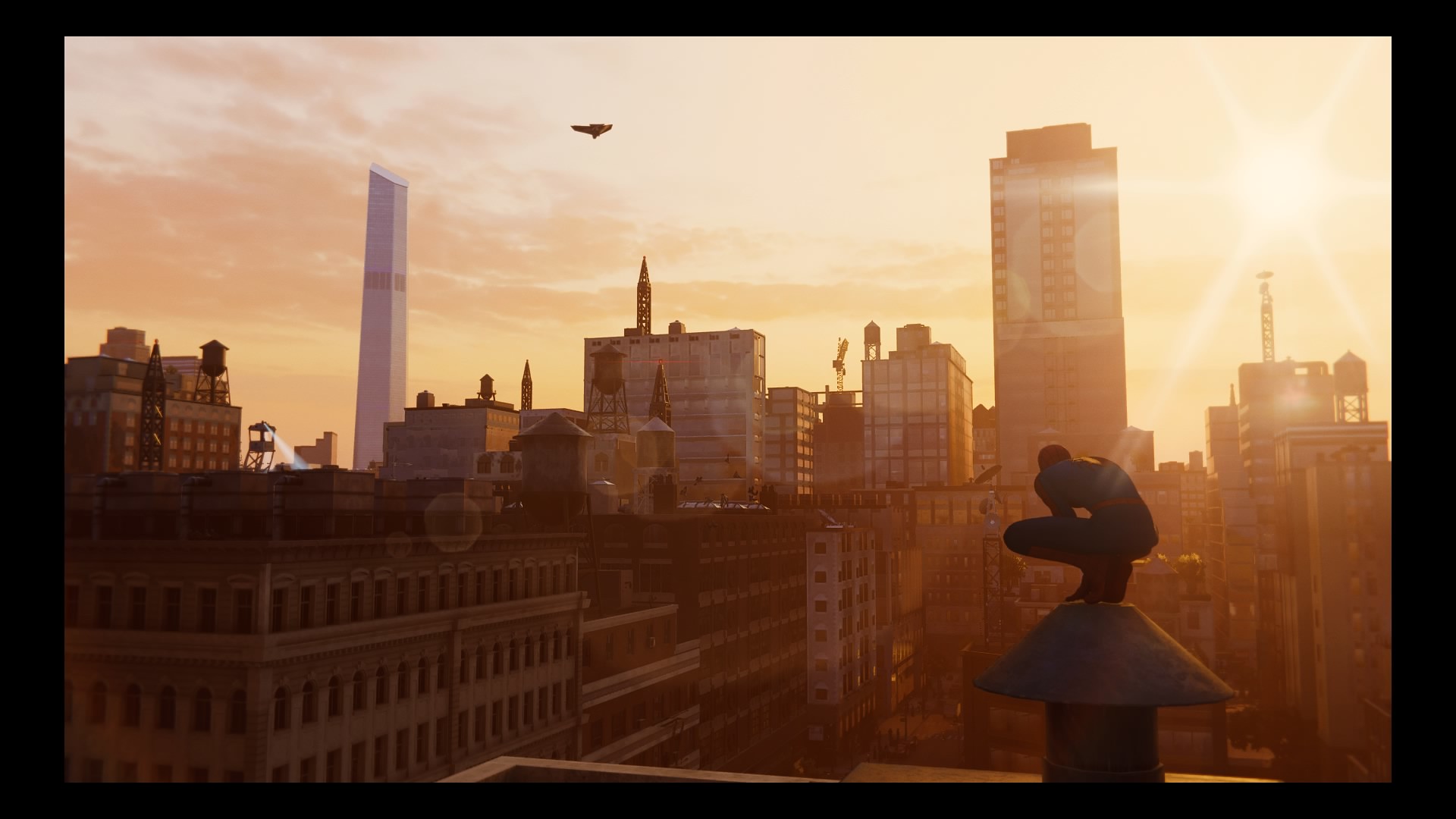In this detailed image capturing a quintessential New York City scene, Spider-Man is prominently featured, crouched atop a chimney or vent positioned in the bottom right corner of the photograph. The perspective is from the top of a building, granting a sweeping view of numerous other buildings that populate both the foreground and background, defining the iconic New York skyline. Spider-Man's pose suggests he is intently gazing into the distance, possibly at a building or point of interest far off. Taken in the middle of the day, the bright sun high in the sky casts a warm, orange and yellow hue across the scene, though there is some haziness suggestive of afternoon or early evening, adding a soft ambiance to the cityscape. The image, which is rectangular with a left-to-right orientation, is bordered by a black frame, lending a framed, almost computer-generated quality to the photograph. The details within the city, from the varied architecture of the buildings to the possible presence of a bird high in the sky, contribute to the richness of the scene. At the street level, hinted at the bottom of the image, the bustling life of the city is subtly implied.